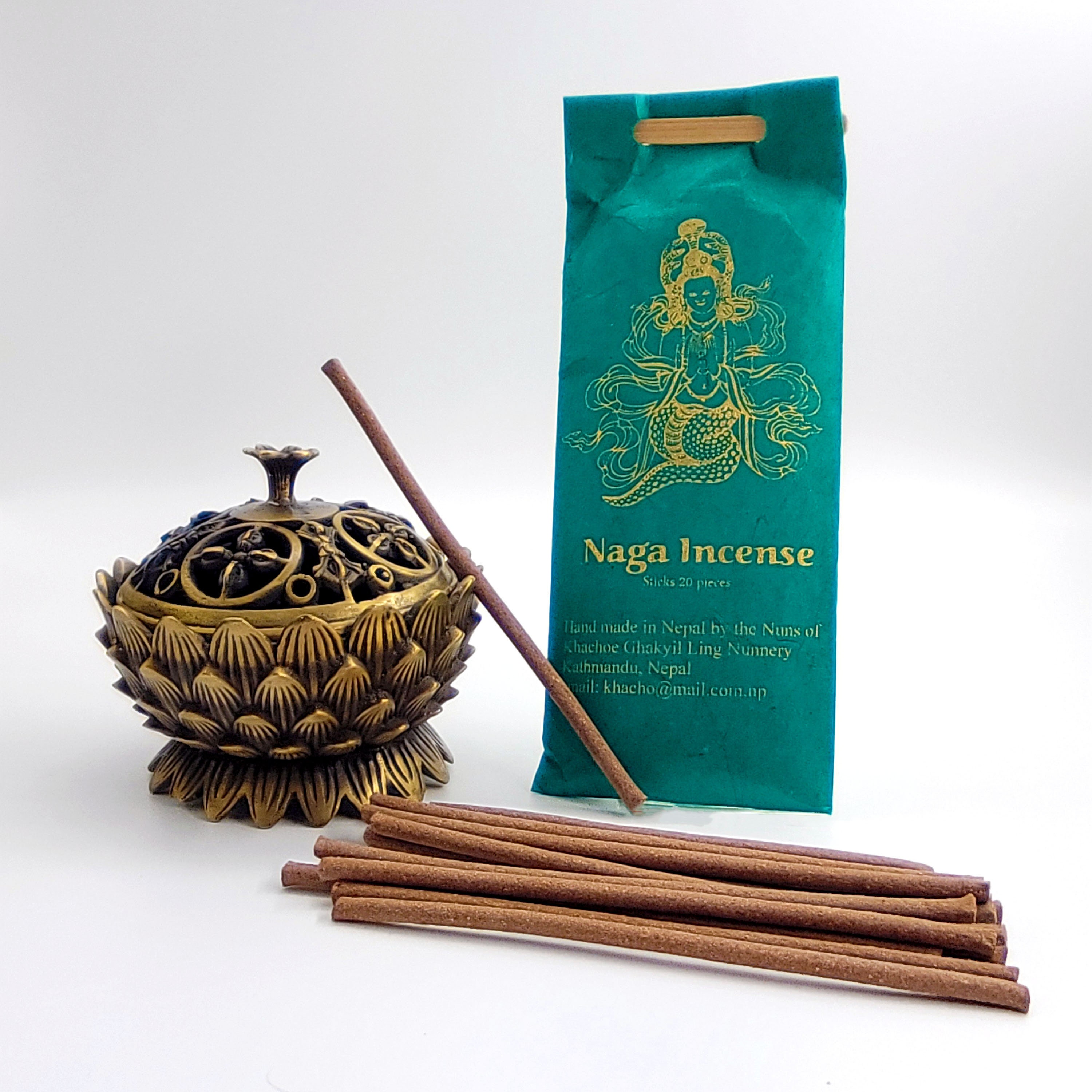The photograph features an elegantly arranged display of incense sticks, their packaging, and a small incense holder, presented against a pristine white background. The long, thin, brown incense sticks lie neatly in the forefront, reminiscent of cinnamon sticks in their linear form. Behind them stands a teal packaging adorned with ornate gold lettering that reads "Naga Incense," accompanied by a sophisticated logo. The package features a detailed illustration of a mermaid-like figure with a fish-tail lower body and intricate hair design, noted as being handmade in Nepal by nuns. To the left of the package is an exquisitely ornate gold incense holder, designed with a petal-like, almost lotus flower shape, and detailed with floral patterns. One of the incense sticks is poised, leaning gracefully against this holder. The overall composition suggests a professional advertisement or catalogue image, highlighting the product's elegant and artisanal qualities.